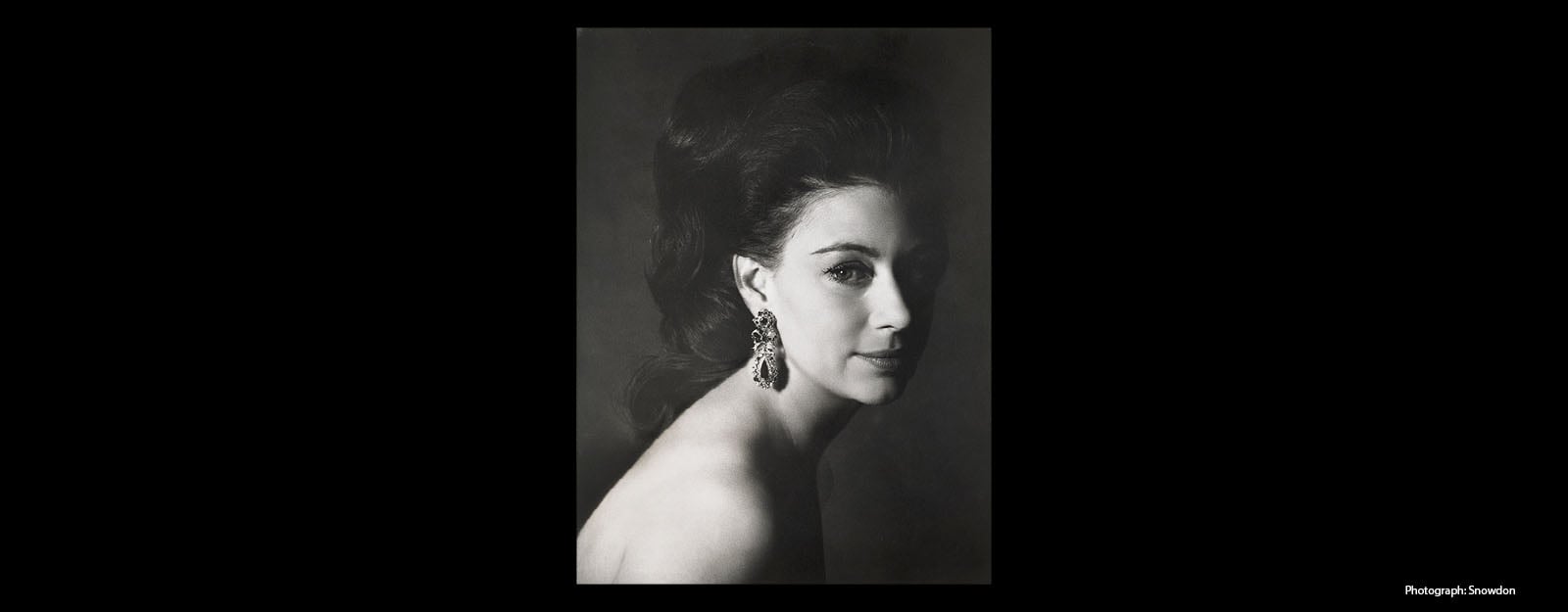The image is a horizontally rectangular black-and-white photograph set against a wide, black background. At the center is a vertically rectangular black-and-white portrait with a gray backdrop. The photograph, signed "Photograph Snowdon" in the lower right corner, features a modern and elegant depiction of a Caucasian woman. She is standing in profile, turning her head to look directly at the camera, with one side of her face in shadow. Her facial features, including her eyes, nose, lips, and chin dimple, are clearly visible. The woman has dark, wavy hair styled in a high, voluminous bouffant that cascades down the middle of her back. She is wearing large, ornate metal earrings adorned with various shapes and black beads, adding to her sophisticated appearance. Although her shoulders are bare, suggesting she may be unclothed from the breast up, the photograph captures only her face and shoulders, leaving her true attire ambiguous. The meticulous composition of the portrait, along with the woman's poised expression, suggests a professionally taken photograph, possibly of an actress or ballerina.